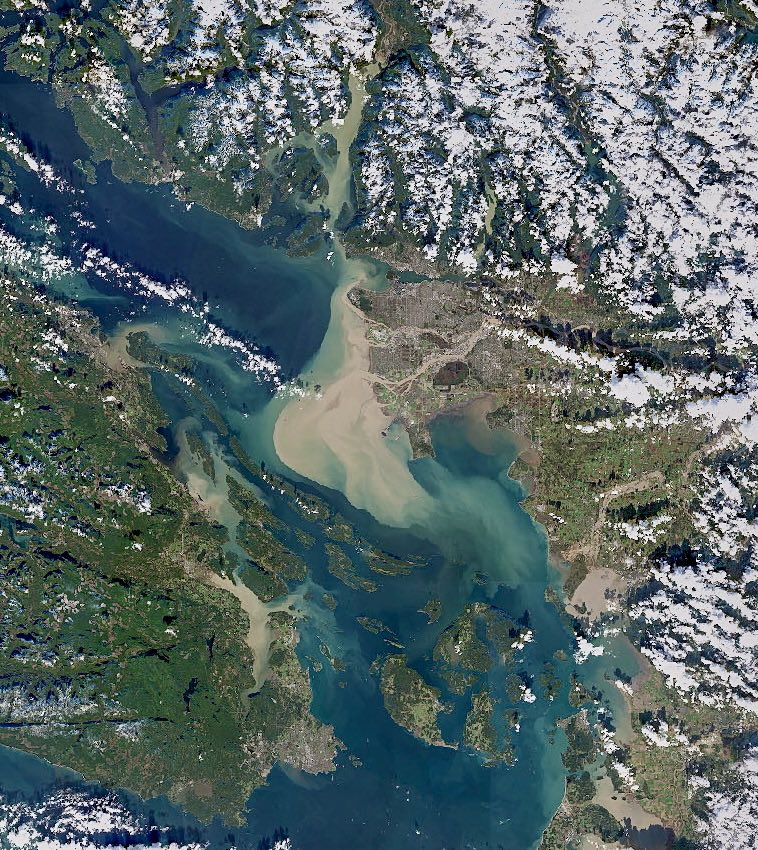This vibrant aerial photograph, possibly taken from an airplane or satellite, captures a scenic top-down view of a picturesque river inlet. The expansive body of water, tinged with light blue and green hues, divides two distinct landmasses. On the right, the landscape is dominated by snow-covered trees or snow-capped mountains stretching towards the upper right corner, imparting a frosty charm. In contrast, the left side is primarily lush and green, punctuated by sparse patches of snow. The central waterway features several small islands and a sandy beach-like area with tan-colored terrain extending from the right. The entire scene, teeming with natural beauty, is enveloped in a serene springtime ambiance with a striking blend of blue water, verdant greenery, and pristine white snow.